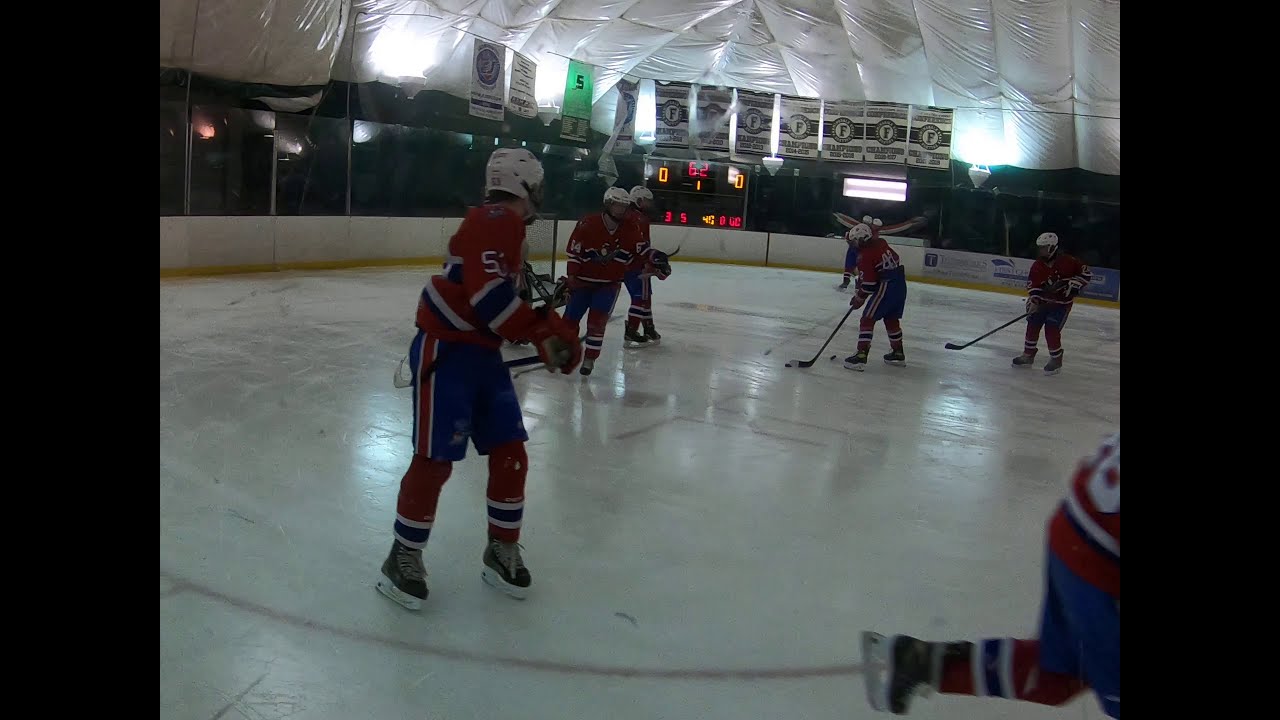This detailed image captures an indoor ice rink featuring several male hockey players, likely from a minor league team, engaged in a practice session. The players are skating energetically, honing their hockey moves and formations. There are about six to eight players on the ice, all wearing red jerseys with blue and white stripes, white helmets, and black ice skates. The rink is surrounded by a white barrier with plexiglass, ensuring safety. The background showcases several banners hanging against the wall; one is notably green with the number 5 on it, while the others are white, possibly commemorating teams or players. Notably, a scoreboard, reading 0-0 and displaying the number 62 in red letters, frames the setting, though it suggests no current game score. The rink area, devoid of spectators, accentuates the focus on practice, with a diminutive yet distinct white-tarp-like ceiling completing the scene.